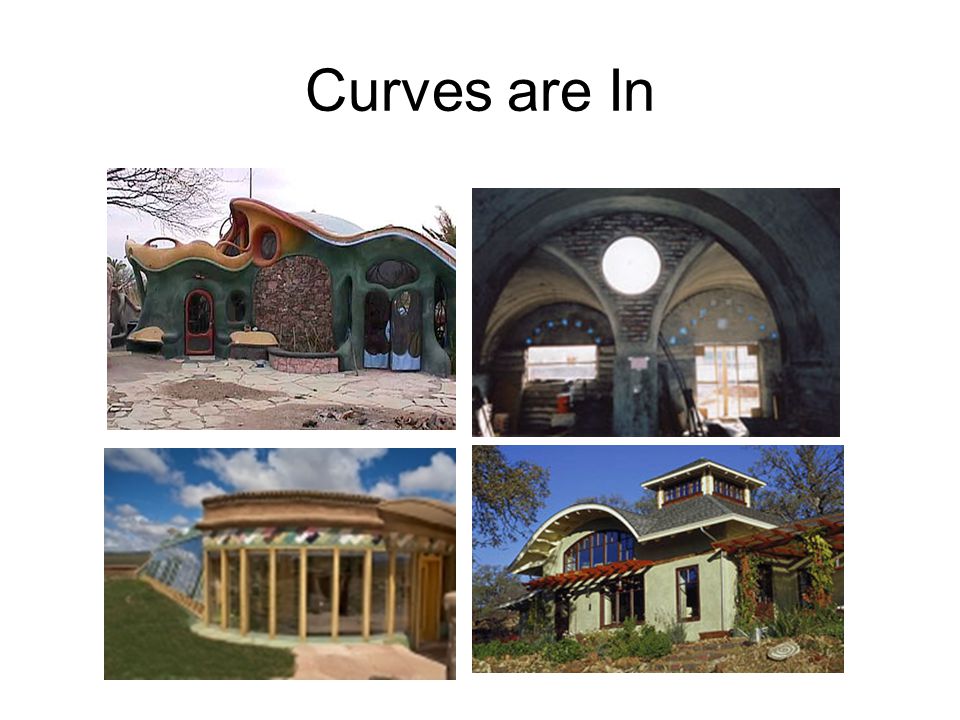The image is a PowerPoint slide titled "Curves Are In" at the top, featuring a collage of four rectangular photographs, each highlighting architectural structures with curved designs. The top section of the slide has a white background with black text, reading "Curves Are In," with the "C" in "Curves" and the "I" in "In" capitalized.

In the upper left, there is a cartoony-looking building with a green exterior, featuring a curvy roof and a brick inlay in the middle, reminiscent of something out of "The Lord of the Rings." To its right, there is a structure showcasing brick archways and unique porthole-like windows, characterized by its dark gray architecture. 

The lower left of the collage displays a coliseum-like building with large columns and a curved shape, surrounded by green grass and set against a cloudy sky. Finally, the lower right image depicts a typical house with a light green facade and a prominent curved roof section above the windows, complete with a tower-like structure on the right-hand side, bluish windows, a red roof, stairs, and grass in the foreground, with trees and a clear blue sky in the background.

All four pictures emphasize the theme of curvy architectural elements, aligning with the slide's overarching message that "curves are in."